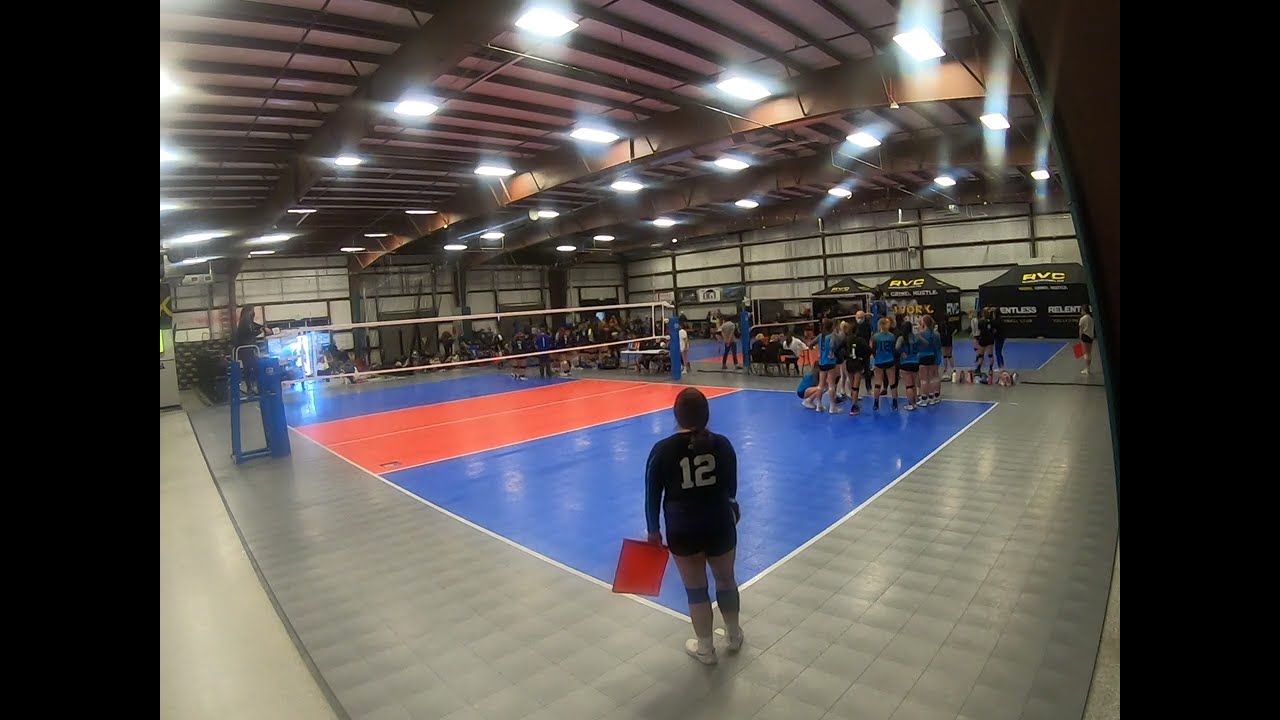This detailed photograph captures the full scene of an indoor volleyball game during a break. The rectangular volleyball court features a vivid blue floor with a red section in the middle, bordered by white lines. A white net divides the court in the center where an umpire is seated. The scene is framed by a gray walking area that extends outward in a V-shape from the perspective of the viewer positioned at one corner of the court. Standing prominently at the lower center of the image is a girl wearing a dark blue shirt and black shorts, holding a red flag and an orange folder. Her shirt has the number 12 printed on the back, and she stands with her back to the camera, observing the court. The players, dressed in blue and dark blue uniforms with knee pads, are gathered in groups, indicating a break in the game. The ceiling above is beige, adorned with wooden beams and multiple bright white lights. Tent-like black structures with writing on them line the far wall of the gym, adding depth to the background where another game appears to be taking place on an adjacent volleyball court.